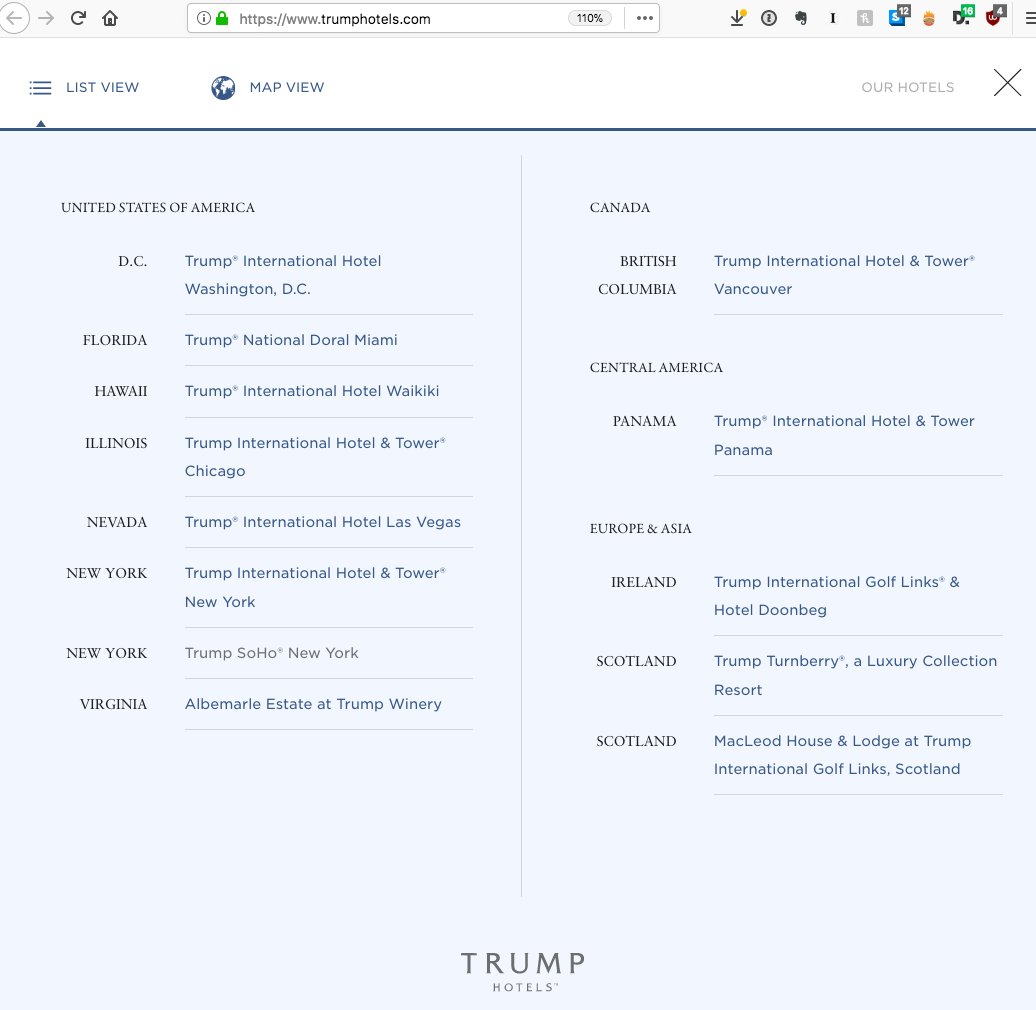The webpage for TrumpHotels.com features a top navigation bar equipped with several icons: left and right-facing arrows, a refresh button, a home button, a download icon, and an information icon. Additional small icons, seven in total, are present but difficult to discern. On the far right of the navigation bar is a hamburger menu.

Below the navigation bar is a white box containing various viewing options, including list view and map view, followed by links to "Our Hotels" and a close button marked with an 'X'. 

The main content area beneath this box highlights various Trump International Hotels across multiple regions:

- **United States of America**:
  - Washington, D.C. - Trump International Hotel, Washington, D.C.
  - Florida - Trump National Doral, Miami
  - Hawaii - Trump International Hotel, Waikiki
  - Illinois - Trump International Hotel and Tower, Chicago
  - Nevada - Trump International Hotel, Las Vegas
  - New York, New York - Trump International Hotel and Tower, New York
  - New York, New York - Trump Soho, New York
  - Virginia - Albemarle Estate at Trump Winery

- **Canada**:
  - British Columbia - Trump International Hotel and Tower, Vancouver

- **Central America**:
  - Panama - Trump International Hotel and Tower, Panama

- **Europe and Asia**:
  - Ireland - Trump International Golf Links and Hotel Doonbeg
  - Scotland - Trump Turnberry Luxury Collection Resort, including McLeod House and Lodge at Trump International Golf Links

At the bottom of the page, the Trump Hotels branding is displayed prominently.